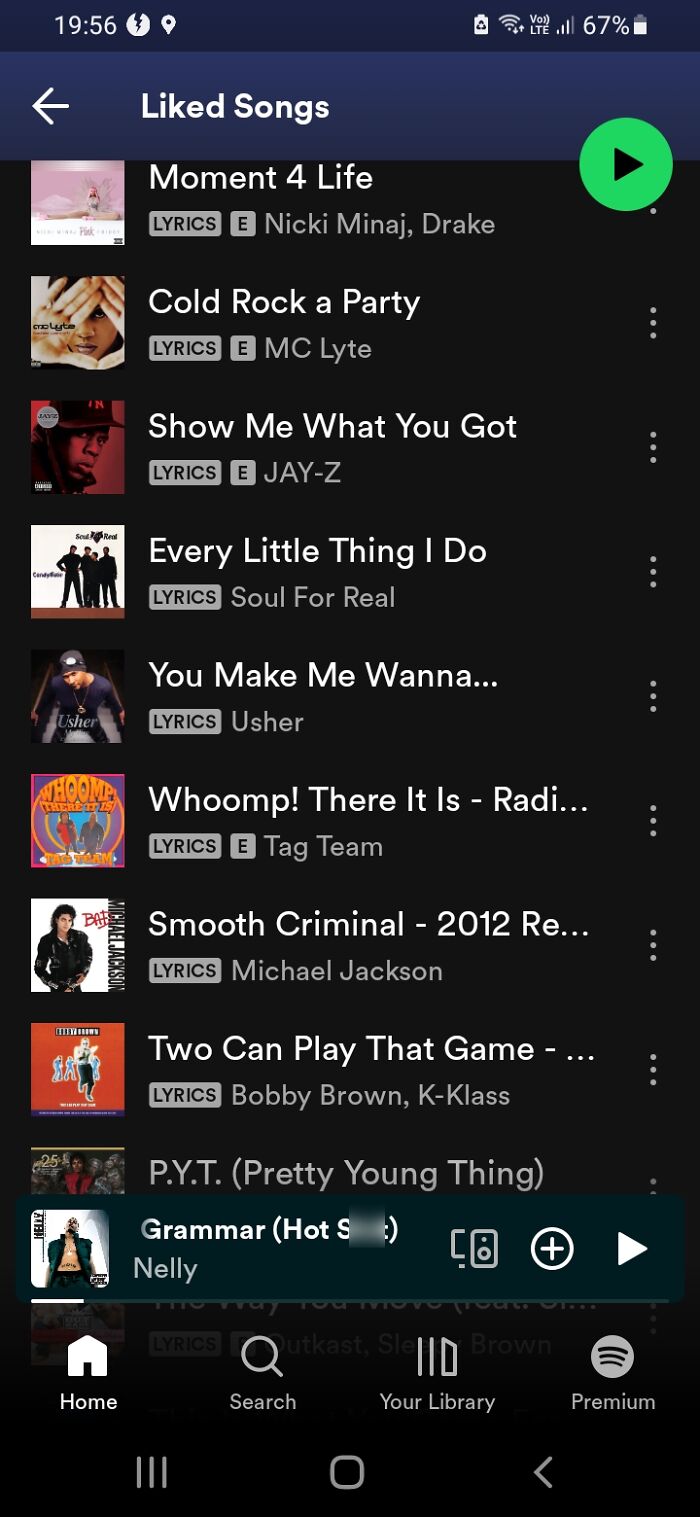The image captures a screenshot of a smartphone screen displaying a playlist titled "Liked Songs." At the top of the screen, standard phone icons are visible, including battery status, signal strength, and possibly Wi-Fi or cellular connection indicators, all set against a predominantly black background. Just below these icons, a blue banner with white text reads "Liked Songs" and features a navigation arrow pointing to the left, indicating the option to go back to a previous screen.

The main portion of the screen displays a list of approximately ten songs, each likely representing an individual track that the user has marked as liked. The songs are organized in a vertical list format. To the left of each song title, there might be icons or thumbnail images representing album covers or artist photos.

At the bottom of the screen, a row of navigation icons is present for quick access to different sections of the music application. These icons include options for Home, Search, Your Library, and Premium. Additionally, a prominent green play button is located near the song listings, indicating the option to play the selected playlist or individual songs. The overall interface is sleek and user-friendly, designed to facilitate easy music selection and playback.